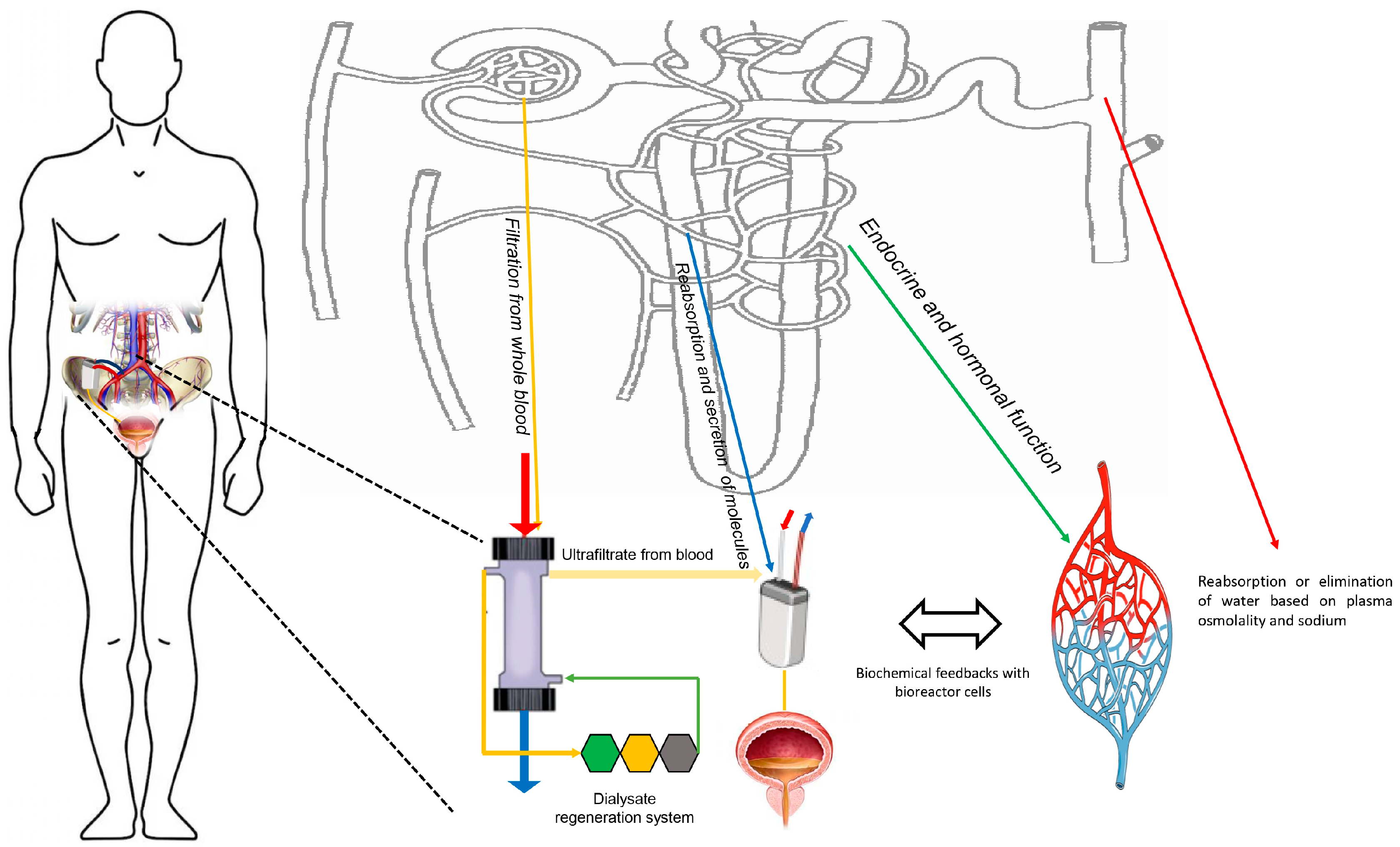The image presents a comprehensive and detailed diagram of the dialysis process within the human body, focusing primarily on the kidneys and the renal system. It outlines the body, particularly around the pelvic region, depicting the kidney's role and the corresponding dialysis system. The diagram features nodes, arrows, and descriptive labels that illustrate the blood filtration process, highlighting stages such as filtration from whole blood, ultra-filtration, dialysate introduction, and reabsorption or elimination of molecules and water. Key elements include biochemical feedbacks with bioreactor cells, endocrine and hormonal functions, and regulatory mechanisms involving plasma osmolality and sodium. The left section emphasizes blood ultrafiltration, while the right details water treatment. Red and blue leaf-like shapes within the image symbolize different aspects of the filtration process. For more detailed information, visit www.FEMA.gov.